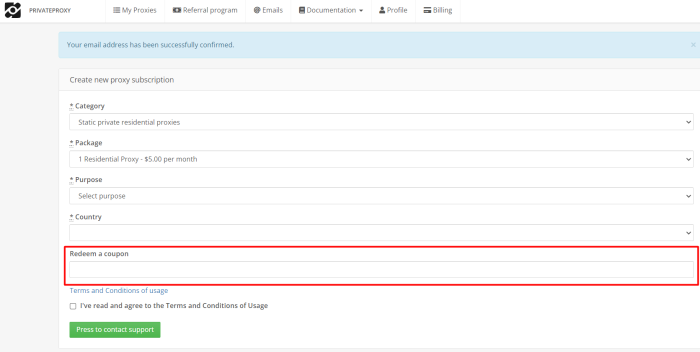The screenshot displays a page from the "Private Proxy" website. The "Private Proxy" title is prominently positioned in the upper left corner, accompanied by the company's logo. The logo consists of a small black box featuring a pattern of circles and lines in its center. Along the top navigation bar, several tabs are visible, including: "My Proxies," "Referral Program," "Emails," "Documentation," "Profile," and "Billing."

The main content area begins with a light blue notification bar at the top, indicating that the user's email address has been successfully confirmed. Below this notification, there's a section labeled "Create a New Proxy." Lower on the page, a text field within the "Redeem a Coupon" section is prominently highlighted with a red square outline, though the field itself is currently empty.

Beneath the "Redeem a Coupon" section, there's a statement titled "Terms and Conditions of Usage," accompanied by a checkbox for users to affirm they have read and agree to the terms and conditions. Finally, in the bottom left corner, a green button labeled "Press to Contact Support" is available for users needing assistance.